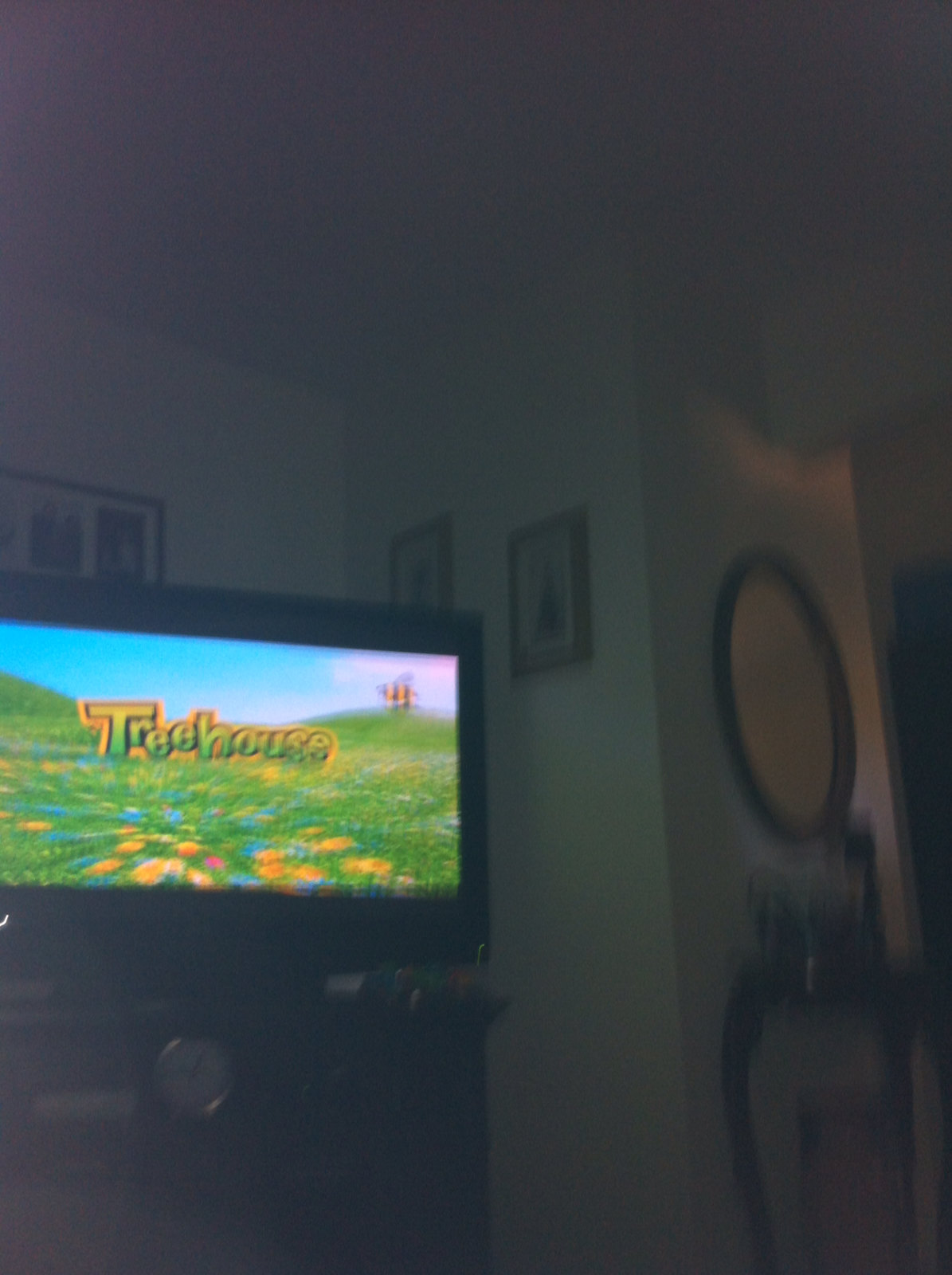The image depicts a somewhat darkened room, taken from the perspective of an unseen viewer watching television. The focal point is a flat-screen TV positioned on a dark nightstand or table, showing a children's program labeled 'Treehouse' in green and yellow outlined letters against a background of a blue sky, rolling green hills, and white puffy clouds, with flowers and a cartoon bee visible. The room's off-white walls feature three framed pictures: one directly behind the TV on the left and two more on the right wall. To the right side of the scene is a dark brown round mirror mounted above a small, spindly-legged table. A white partition extends from the ceiling outward from the wall, adding to the room's layout. The overall aesthetic suggests a slightly blurry, cozy living room environment.